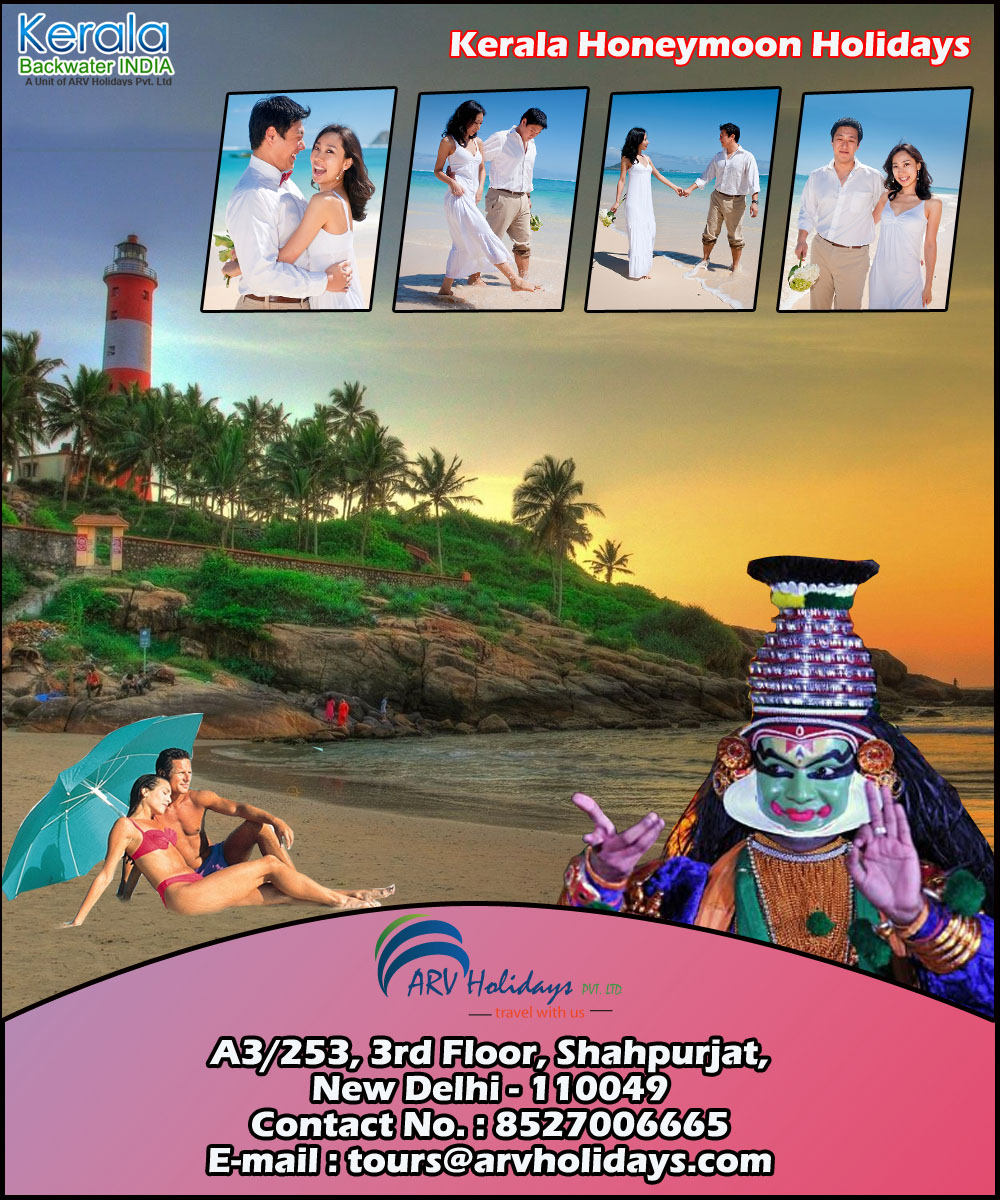A vibrant full-color print advertisement showcases a serene tropical beach scene at either dawn or dusk. The pristine sandy shore gently meets the crystal-clear water, creating a tranquil setting. A lush hill rises in the background, adorned with verdant green plants and graceful palm trees swaying in the breeze. At the hill's summit stands a striking red and white striped lighthouse, adding a picturesque focal point to the landscape. 

In the foreground, superimposed on the beach, a couple can be seen enjoying the serene environment. She is wearing a bikini, while he is dressed in blue pants; they are lounging comfortably under a blue umbrella, savoring their moment of relaxation. Adding an intriguing element to the scene, an ethnically distinct entertainment character is also superimposed, bringing a unique and eye-catching aspect to the advertisement.